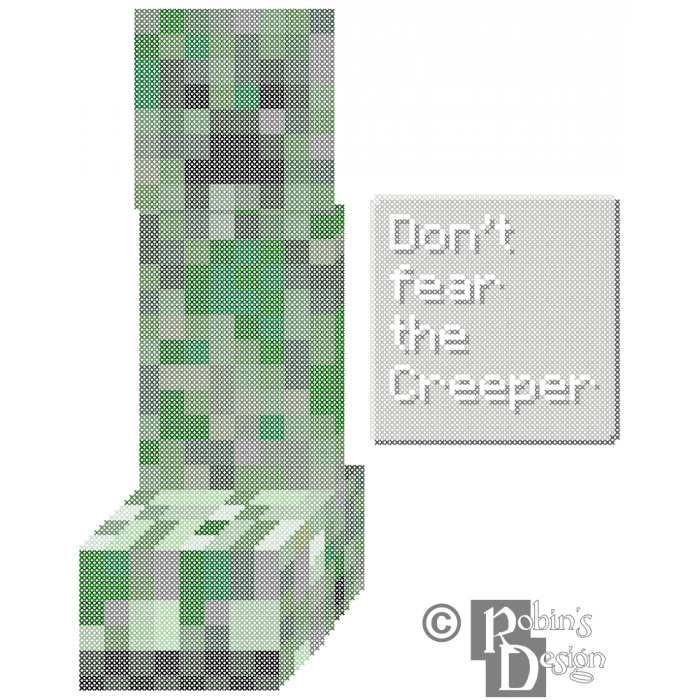The image is an advertisement featuring the text "Don't Fear the Creeper" in white, pixelated font set against a gray background square. To the left of the text, there is a pixelated figure reminiscent of Minecraft characters, constructed from small squares in shades of green, gray, and camouflage-like patterns. The figure has a thinner upper section—representing the head—and a thicker lower base, evoking the distinct blocky style of Minecraft. At the bottom right corner of the image, there is the phrase "Robbins Design" accompanied by a copyright symbol, neatly placed within a small black box on a white background, deviating from the pixelated theme. The entire composition also rests on a white background, providing a clean contrast to the pixelated central elements.